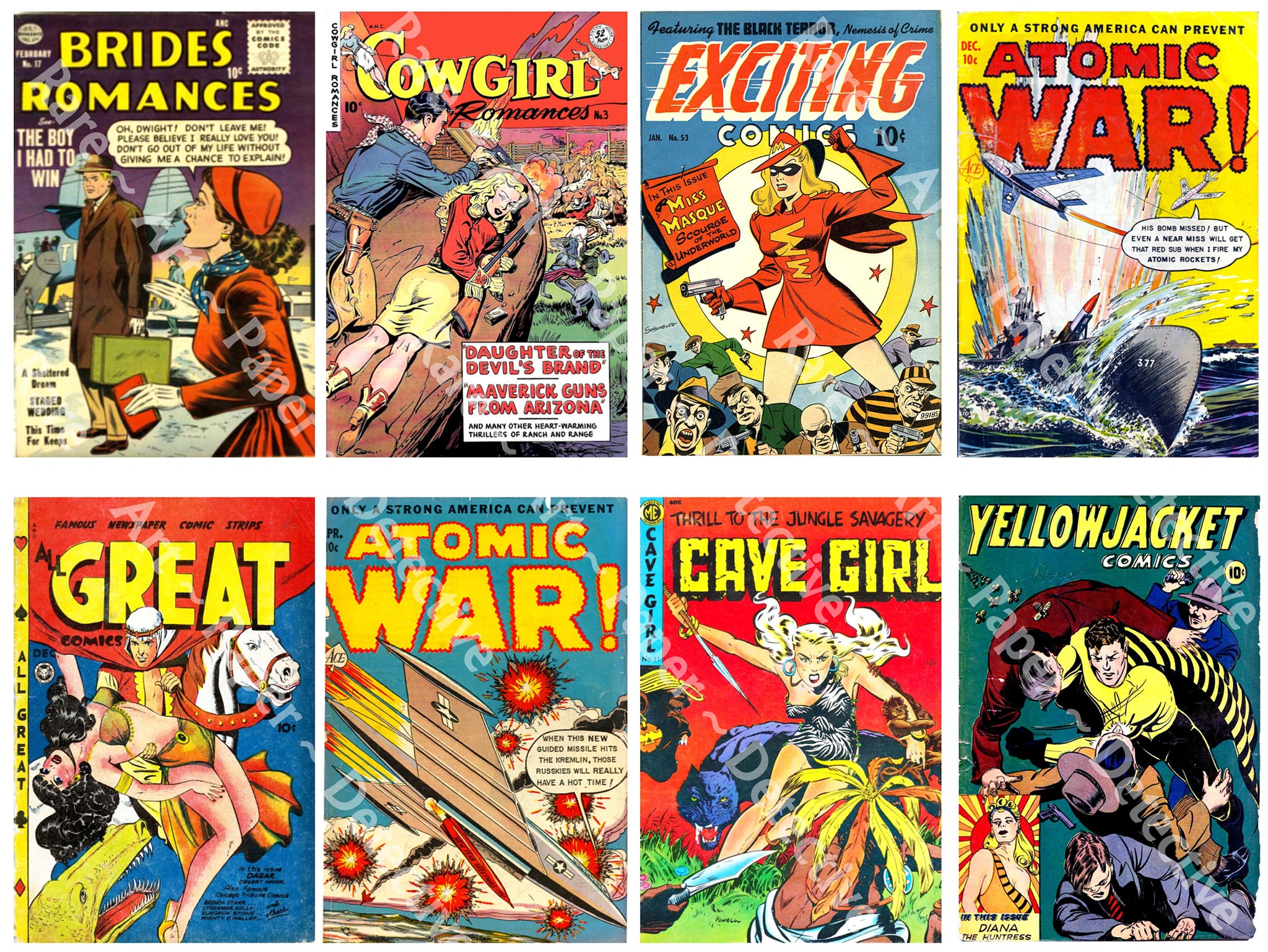The image is a meticulously arranged collection of eight vintage comic book covers from the 40s, 50s, and possibly the 60s, presented in two rows of four. The vibrant colors of the covers include bright yellows, reds, blues, and greens. Each cover features bold titles in yellow or red letters. Starting from the top left, the first cover is "Brides Romances," depicting a pleading woman in a red dress next to a man in a brown overcoat. The next cover, "Cowgirl Romances," is followed by "Exciting Comics," which showcases a woman in a red dress with a dark mask over her eyes. The top right cover "Atomic War" features planes flying over a ship armed with missiles. Moving to the bottom row, the first cover is titled "Great Comics," illustrating a heroic man with a red cape on a white horse holding a woman in a golden dress. Adjacent to it is another "Atomic War" cover portraying a dynamic scene with a plane and explosions. The second from the right displays "Cave Girl," presenting a woman in a zebra-print outfit, white hair, and a black panther. Finally, the bottom right cover, "Yellowjacket Comics," features a superhero in a yellow and black costume accompanied by other characters in business attire. The comic book covers are spaced evenly, forming a neat and nostalgic grid.